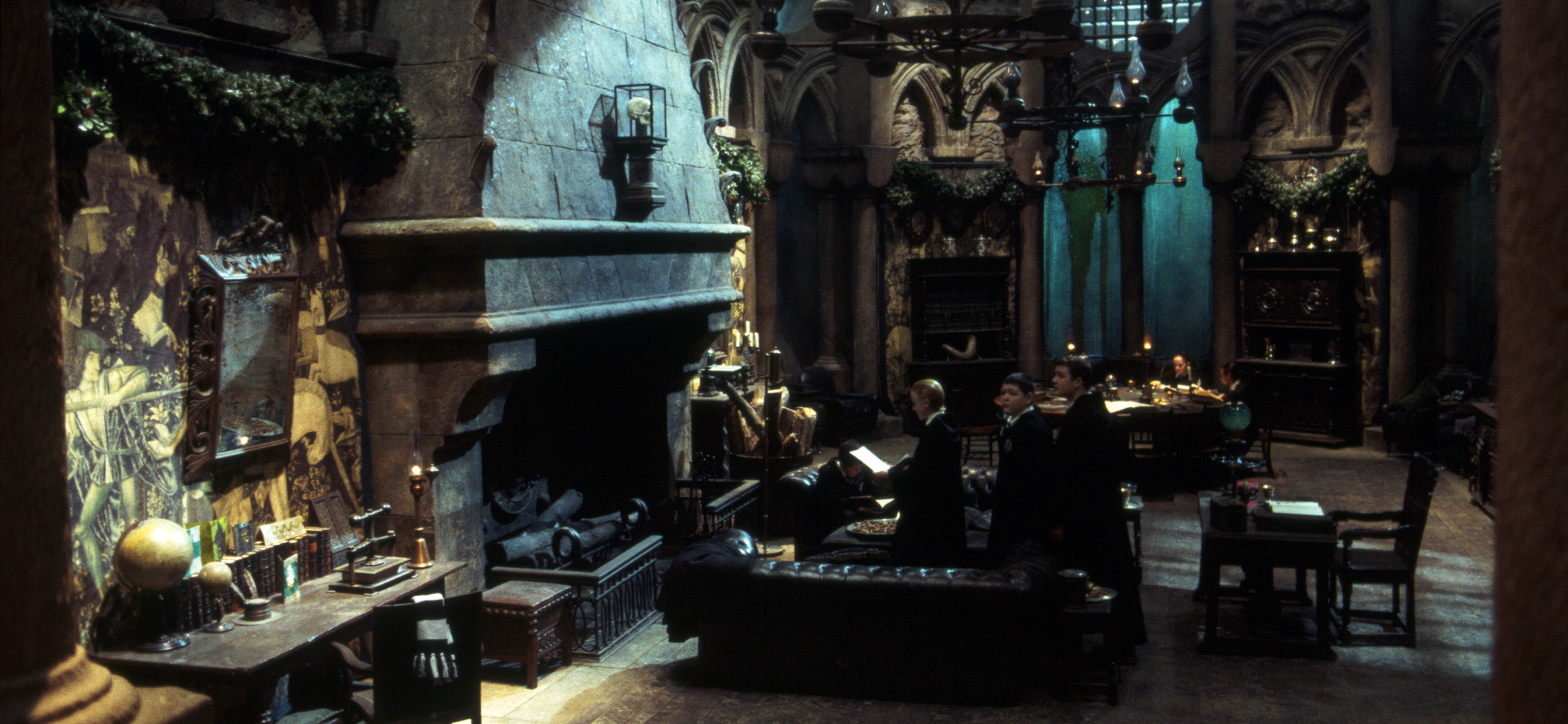The image depicts a dimly-lit scene from a Harry Potter movie, likely set in a medieval-style, underground or basement location. The ambiance is very dark, with gothic architectural elements dominating the scene. In the middle, a large, gray stone fireplace with burnt wood and a gothic metal fence stands out, topped by an antique light featuring a skull inside, but the light is not lit. Flanking the fireplace is a wooden bench with a leather seat and a dusty wooden desk holding various objects, including a yellowish-brown globe and a paper. A Christmas vine wreath hangs on one wall, with a large, indistinct black-and-white painting nearby. The walls are richly carved wood, and there's a tall, dark window, adding to the eerie atmosphere. The floor is covered by a brownish rug. 

Several students in black robes and white shirts, characteristic of Hogwarts attire, are present. One is holding a book or paper, two others are standing, and another is seated on a black leather couch. In the background, there's a dining table with more students studying. A mirror and a pillar are also visible, contributing to the gothic, castle-like ambiance. Despite some sporadic lighting, the overall scene remains very dark and shadowy, enhancing the movie's mysterious and suspenseful mood.